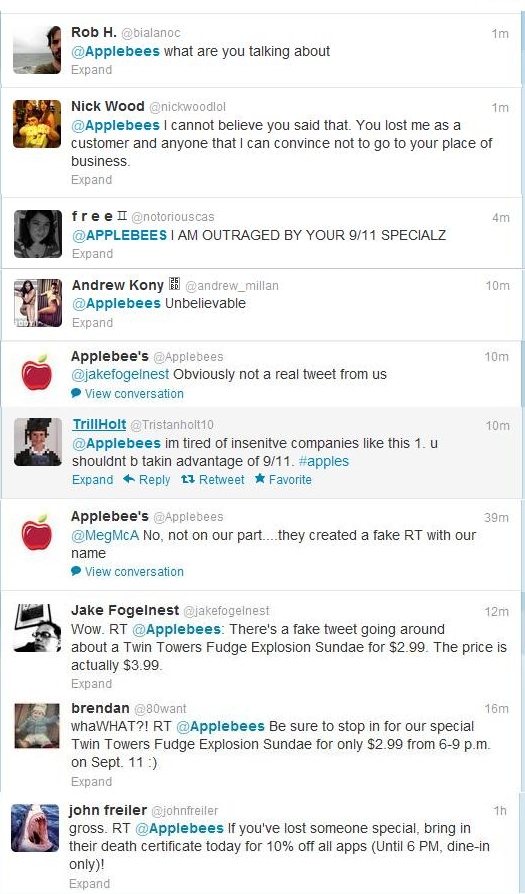The image displays a social media feed, likely from Twitter or X, featuring a heated discussion involving the Applebee's restaurant chain. The background is predominantly white, with text in black font and several user profile pictures included. At the top, Rob H. questions, “At Applebee's, what are you talking about?” followed by Nick Wood’s outraged response, “I cannot believe you said that. You lost me as a customer and anyone that I can convince not to go to your place of business.” Several other users, including Andrew Connery and Trill Holt, express their disdain, particularly about a reportedly insensitive 9/11 special. Applebee's attempts to clarify by responding to Jake Foggenrath and Meg MCA, stating that the offensive tweets are fake. Despite this, more tweets appear, including Brendan's promotion of a "Twin Towers fudge explosion sundae for $2.99," which John Fraylor condemns, calling it “gross.” The theme colors include a deep turquoise with red apple icons beside some entries, possibly signifying the official responses. Overall, the feed reflects a significant backlash against Applebee's, with individuals tagging the company to express their frustration and disbelief over the insensitive promotions.